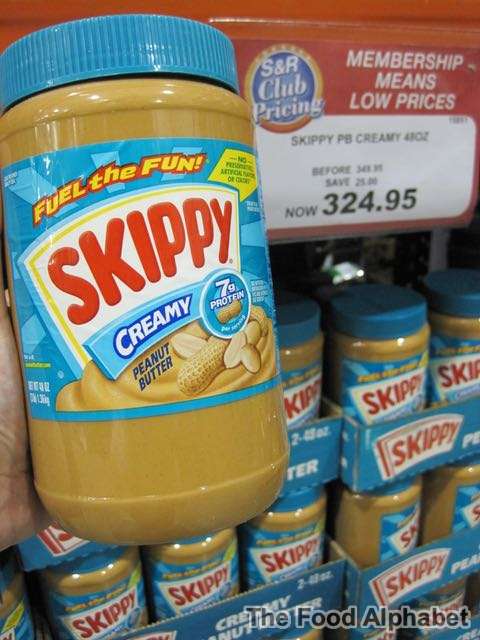Close-up image of a store shelf, prominently featuring multiple jars of Skippy creamy peanut butter. The shelf, painted red, displays the slogan "Membership Means Low Prices" in bold white lettering. A price label, marked in black on a white background, reads: "Skippy Peanut Butter Creamy 48 ounces. Now $3.24.95." The jars of Skippy peanut butter are uniform in design, featuring blue lids and blue labels with the brand name "Skippy" displayed in striking red letters on a white background. The neatly arranged jars create a visual repetition and emphasize the product's availability and discounted price.